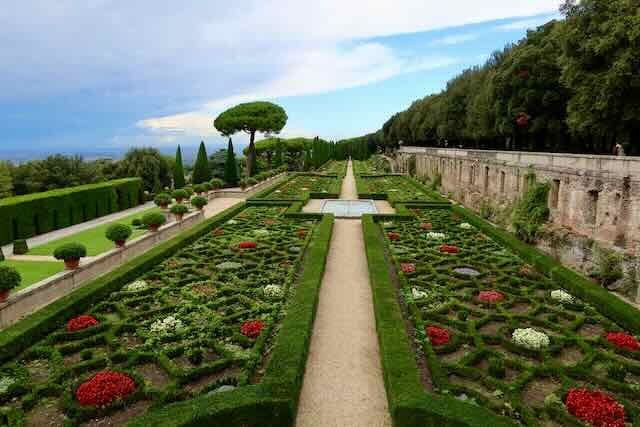The photograph captures an ornate, meticulously designed garden bathed in daylight. The central focus of the image is a geometric, plantar arrangement featuring lush greenery interspersed with vibrant red and white flowers. The garden stretches out along a concrete walkway that meanders through the scene. On the right side of the image, there is a lengthy brick or stone wall with large, mature trees and bushes standing behind it, forming a dense backdrop. The left side of the photograph showcases another shorter stone wall adorned with potted plants that contain flourishing bushes, providing neat, patterned hedges. Clustered around the garden’s center, there is a small, square pond nestled among the flowers and grass. More greenery and trees populate the far left and the horizon, completing the idyllic setting under a blue, cloud-dotted sky. Striking details such as the combination of well-maintained shrubbery, vibrant floral patches, and surrounding walls create a picturesque, almost regal atmosphere that could easily be mistaken for an esteemed estate or historical garden.